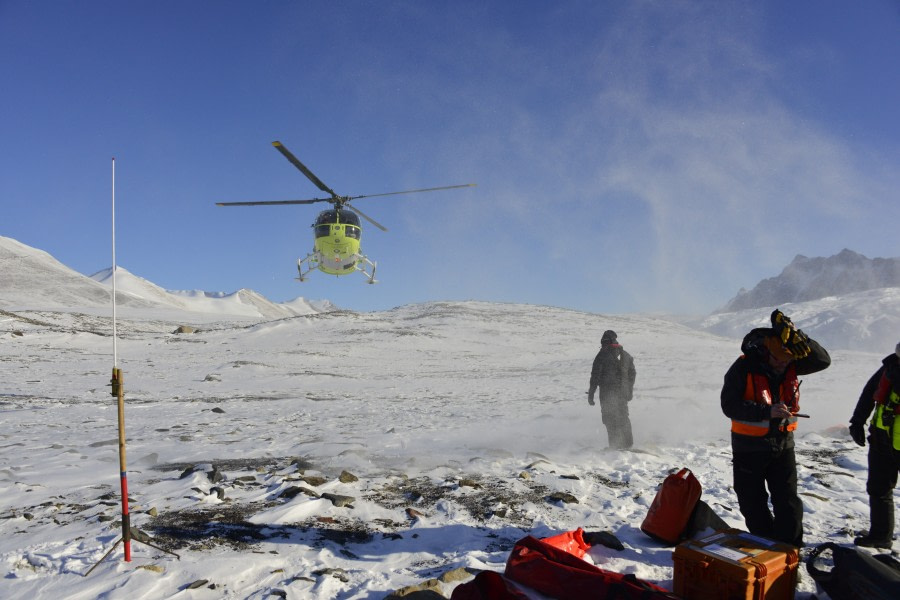The image captures a stark and frigid landscape, possibly in Antarctica, under a clear, bright blue sky. Dominating the scene is a light yellow helicopter with black blades, mid-descent onto a snow-covered hill, its spinning blades kicking up a flurry of snow, creating a mist-like effect. In the right corner stand three individuals clad in thick, dark winter gear, engaged in various activities among their equipment. One faces the helicopter, observing its approach, while the second individual, wearing a neon orange vest, looks down at something in his hands. The third person, partially visible, sports a yellow vest. Scattered before them are several plastic boxes, red bags, and other gear, possibly including supply crates or tents. A red and tan pole, likely a measurement post, is embedded in the snow to the left. The vivid colors of the outfits and helicopter contrast sharply with the pristine white snow and the deep blue sky, creating a visually striking and detailed tableau of a remote, icy environment.